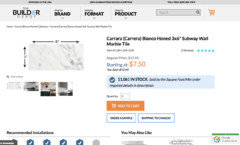The screenshot depicts a shop webpage for "The Builder" with a light gray header. On the top left, the logo reads "The Builder" with the word "Builder" in black except for the letter "E," which is in a curved blue font. Adjacent to the logo are dropdown options for "Brand," "Format," and "Product," each accompanied by a blue downward arrow. To their right, there is a medium gray search bar displaying the word "Search" and a magnifying glass icon. An orange shopping cart icon is positioned at the far right.

The main section of the webpage has a white background, featuring product images on the left and product information on the right. Though slightly blurry, the primary product image shows a rectangular object, likely a marble countertop or similar material, with measurement arrows pointing horizontally and vertically. Underneath this main image are four smaller images—two square ones on the right and two rectangular ones on the left—offering different angles of the product, although the details are indistinct.

To the right of these images, the product information includes a bold black title ending with "Marble Tile," though the preceding text is unreadable. A blue star rating, appearing to be a five-star rating, is situated below and to the right of the title. Additionally, an orange price tag indicates "Starting at $7.50," with the dollar amount in orange and the phrase "starting at" in blue.